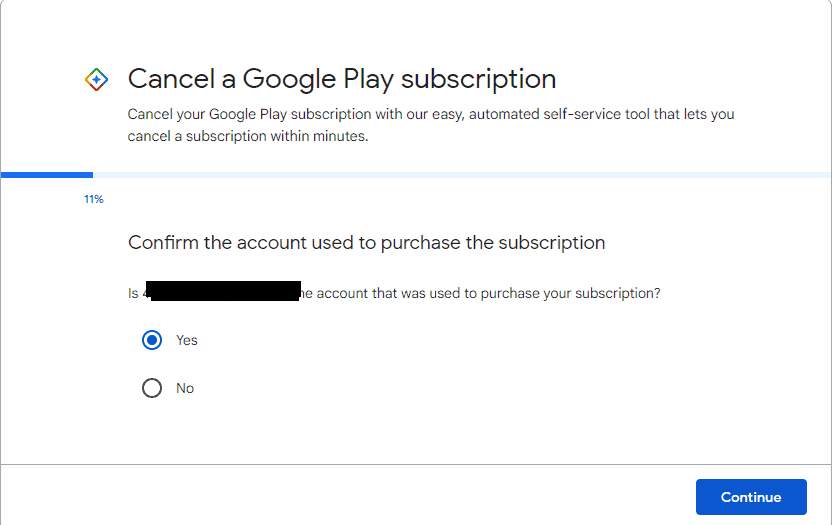The image, sourced from Google, features a white background and prominently displays a small diamond-shaped insignia adorned with the signature Google colors: blue, gold, red, and green. Adjacent to this insignia, large black text reads "Cancel a Google Play subscription." Beneath this header, a subtext provides further details: "Cancel your Google Play subscription with our easy automated self-service tool that lets you cancel a subscription within minutes."

A horizontal blue progress bar stretches from left to right, indicating that the process is 11% complete. Below this bar, the text instructs the user to "Confirm the account used to purchase a subscription." A portion of this text is obscured by a black marker, but the visible part reads, "Is [blacked out] account that was used to purchase your subscription?"

Options for confirmation are presented as two round, labeled circles: one with "Yes" and the other with "No." A user has selected "Yes," evidenced by a blue-filled circle next to the "Yes" label. 

Below these elements, an empty section is followed by another blue horizontal bar featuring the word "Continue" in white text.